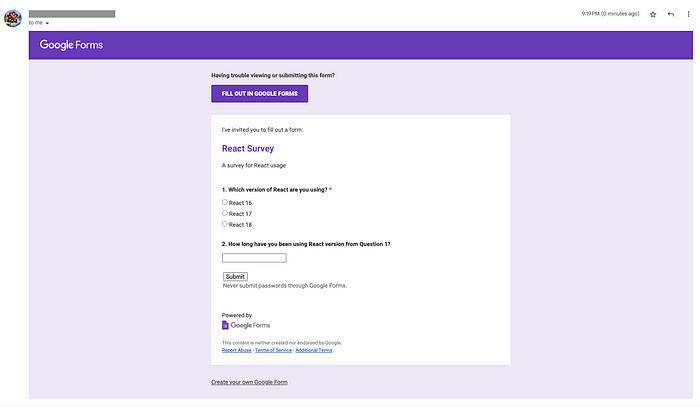The image depicts a Google Forms survey interface. Dominated by Google's signature purple theme, the top bar stretches across the screen from left to right in a darker shade of purple. Centrally placed at the top, "Google Forms" is written in white. An emoji-like image of a flower with a blue sky background is located at the top left above the Google Forms title.

On the top right, the timestamp reads "9:19 PM" with a note indicating it was recorded zero minutes ago, accompanied by a star icon for favoriting, a left arrow icon, and a three-dot menu for additional options.

Directly beneath the "Google Forms" title is a message stating, "Having trouble viewing or submitting this form?" in black text, followed by a prominent purple button labeled "Fill out Google Forms." Below this, the text reads, "I've invited you to fill out a form" in black, with "React Survey" in purple, spaced out beneath it. Further down, it says, "Survey for Reactive Usage."

The first survey question asks which version of React the user is using, provided as a multiple-choice question. 

The second question is a fill-in-the-blank query about how long the user has been using React. 

A "Submit" button is present at the bottom of the form, followed by a disclaimer urging users never to submit passwords through Google Forms. Finally, the form is signed off with "Powered by Google Forms," and the content clarifies whether it was created or endorsed by Google, alongside links to report abuse, the terms of service, and additional terms.